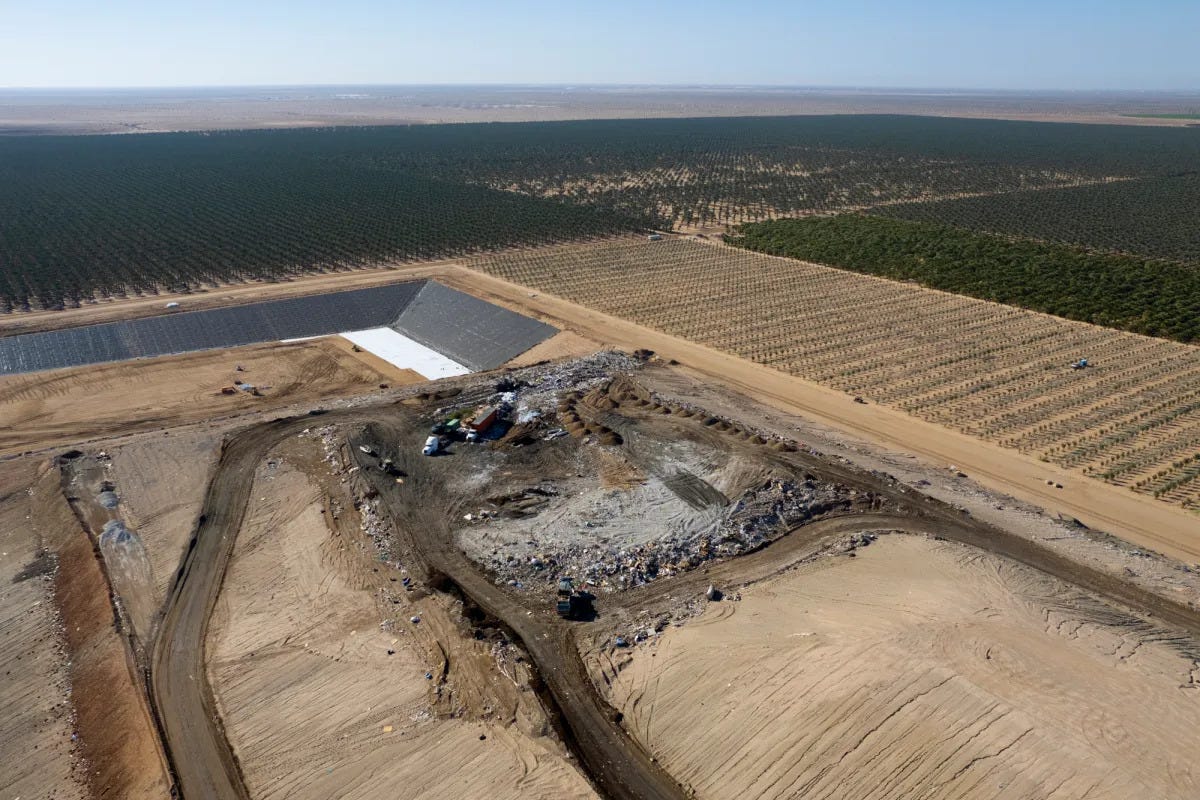This aerial landscape photograph captures a stark and contrasting scene of human activity and natural elements. In the upper portion of the image, three distinct fields of crops stretch across the horizon, separated by light brown rows of soil. The crops are too distant to identify, but their orderly patterns hint at agricultural activity. The background fades into a flat expanse of earth, devoid of greenery, under a thin strip of grayish-blue sky.

In the foreground, the image transitions into a more industrialized and disturbed area. Dominated by large roads and what appears to be a mining or construction site, this section is characterized by scorched and dug-up dirt, with visible debris and dirt paths crisscrossing through it. The site seems messy and chaotic, with small trucks and semi-trucks dotting the scene, leading to piles of dirt and potential runoff areas. There is also an indentation behind the roads, possibly hinting at a lake, a man-made dam, or a concrete container, though its exact purpose is unclear. This part of the landscape contrasts sharply with the organized fields further back, highlighting the varied use of the land.